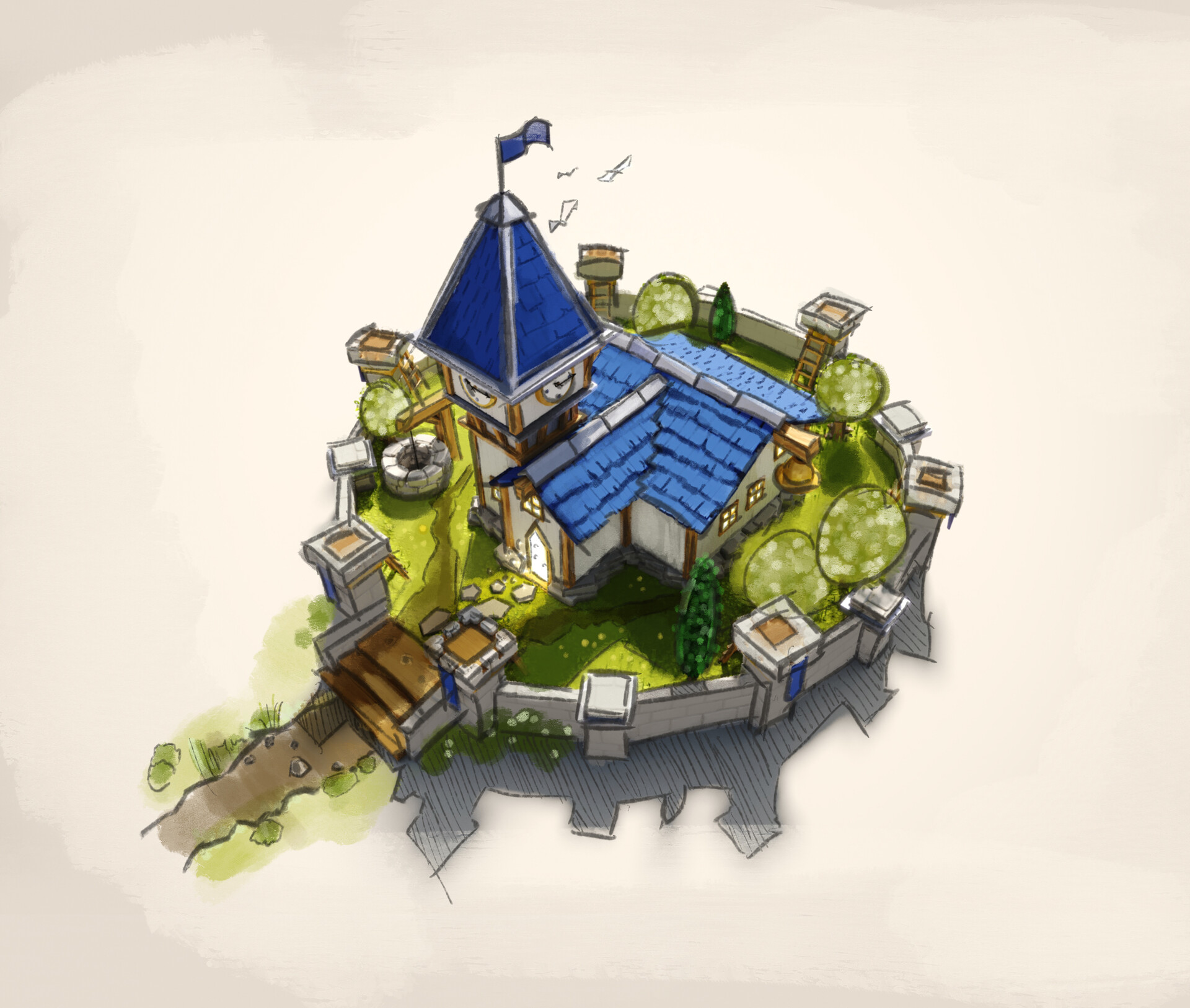The image is a detailed, bright color drawing on off-white parchment, depicting a single, blue-roofed house enclosed within a circular stone gate fence. The house features white walls with timbered corners and a prominent clock tower, which also has a blue roof and a blue flag at its apex. The clock displays faces on at least two visible sides. The building resembles a small castle or church, complete with cobblestone pathways and brown stairs leading to a well-lit door. There is a grassy area with a water well, large trees, and small watchtower-like structures positioned along the fence. Birds can be seen flying overhead, and the sun casts shadows across the scene, suggesting it is daytime. This intricate illustration captures an aerial view of the quaint, enclosed property, creating a whimsical and inviting atmosphere.